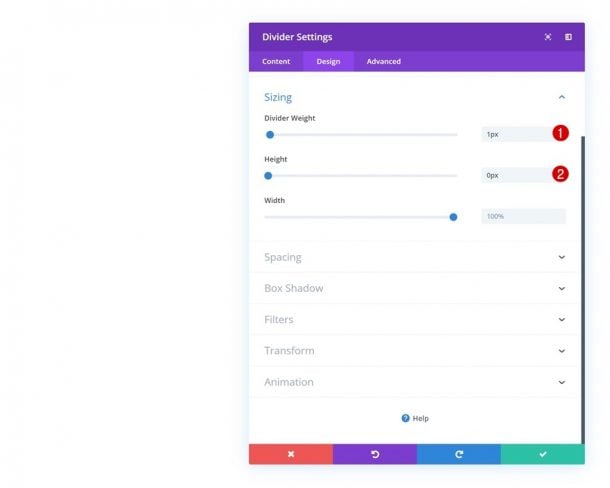This image is a detailed color screenshot in portrait format, evidently taken from a mobile phone, as suggested by its customized dimensions fitting a mobile screen. The screenshot showcases the settings interface for a design feature known as "Divider Settings." At the top of the screen, there are three navigational tabs labeled "Content," "Design," and "Advanced," with the "Design" tab currently selected.

Under the "Design" tab, a suite of adjustable settings is displayed:
1. **Sizing**: Includes a control for "Divider Weight," visually represented by a slider bar, which is currently adjusted to the minimum position on the far left.
2. **Height**: This setting is also set to the minimum value on the far left.
3. **Width**: In contrast, the width is maximized, with the slider fully moved to the right.

Additional customization options available under this tab include:
- **Spacing**
- **Box Shadow**
- **Filters**
- **Transform**
- **Animation**

Below these settings, there is a help button for users needing further assistance. Towards the bottom of the interface, there are three action buttons with distinct colors:
- A red "X" for canceling the changes.
- A purple refresh or back button.
- A green checkmark for proceeding with the current settings.